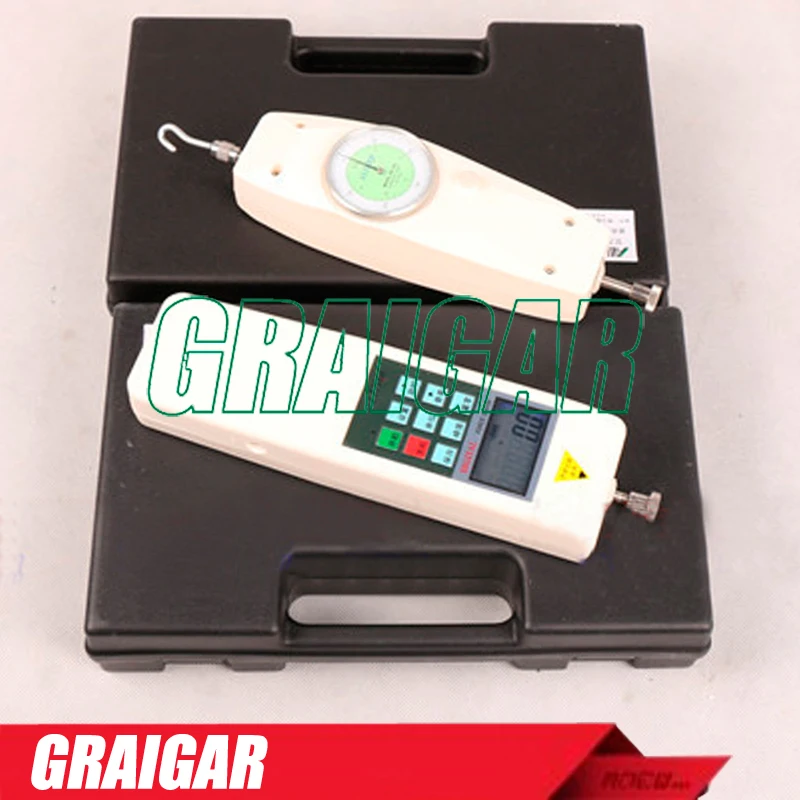The image captures two white, rectangular measuring devices positioned at a diagonal atop two black, hard plastic cases with handles. The upper device, resembling a luggage scale, features a silver hook on top and a dial likely used for measuring weight. Below it, the second device, which has a screen displaying "00" and a 3x3 keypad grid, evokes the look of an old landline phone but is clearly another type of measuring tool. Both devices showcase silver twist mechanisms. The black cases, oriented back-to-back in the image's center, contribute to the industrial, business-like ambiance, further emphasized by the tan off-white background. Green text spelling "GREGAR" overlays the devices, while a red banner with the same name sits at the bottom, suggesting a company logo or watermark.